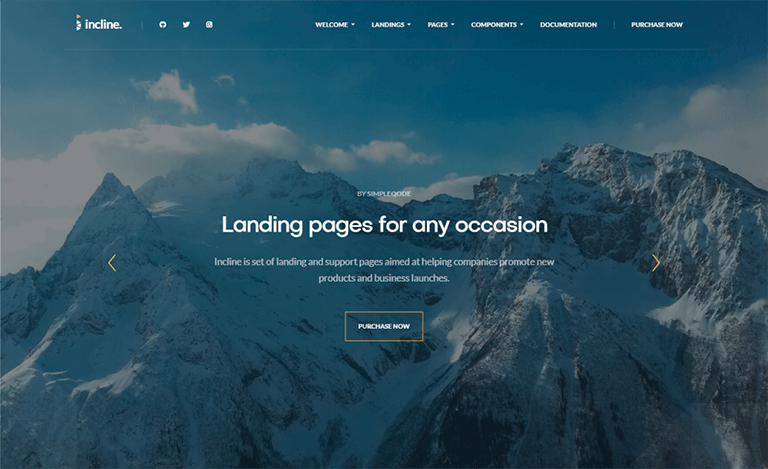This image is a screenshot of a webpage with a visually striking background featuring a snow-covered mountain peak set against a backdrop of a clear blue sky with scattered white clouds. In the upper left corner, a logo reading "INCLINE" in white font is prominently displayed. Adjacent to the logo, social media icons for Facebook, Twitter, and Instagram are neatly aligned, followed by a series of drop-down menus also in white font. These menus are labeled "WELCOME," "LANDINGS AND PAGES," "COMPONENTS," "DOCUMENTATION," and "PURCHASE NOW."

Dominating the center of the image, bold white text declares, "BY SIMPLE CODE, LANDING PAGES FOR ANY OCCASION." This headline is followed by a brief description: "INCLINE is a set of landing and support pages aimed at helping companies promote new products and business launches."

Below this text, a prominent red rectangle outlined in red contains the call-to-action message "PURCHASE NOW" in white font. Flanking this message, red arrows point left and right, adding dynamic visual cues to the call-to-action button. Overall, the webpage combines a striking natural landscape with clear, purposeful text and navigation elements designed to engage visitors and direct them towards purchasing landing and support pages.